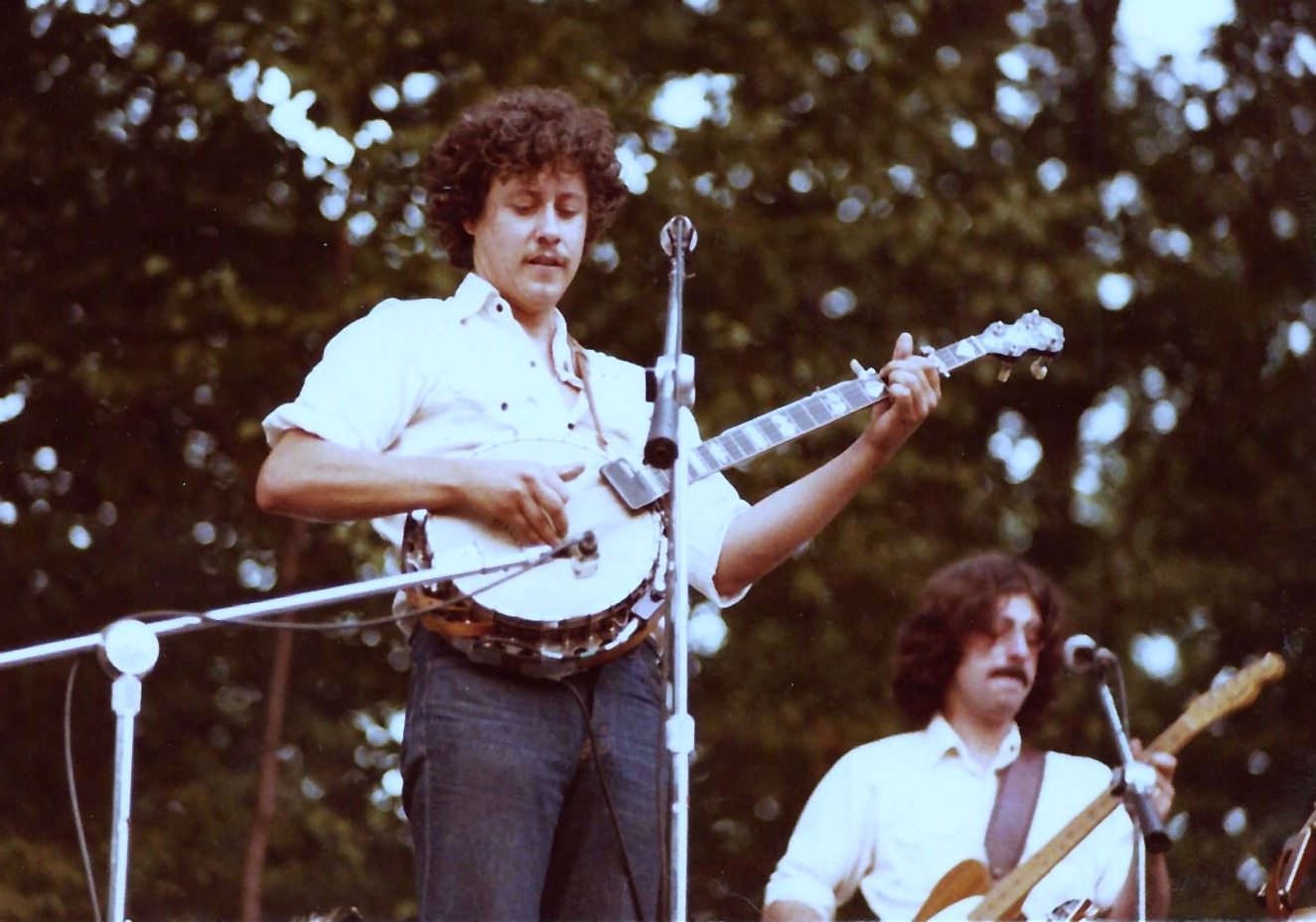This photograph captures a lively outdoor scene where two musicians are performing amidst a backdrop of lush green trees. The man in the foreground, characterized by his curly brown hair and collared white shirt, is strumming a banjo-like instrument with a round, circular body. A microphone stand is positioned in front of him, ready to capture the audio of his performance. To the bottom right of the image, another musician is seen holding a guitar, contributing to the musical atmosphere. Multiple microphone stands are set up around them, indicating a prepared and professional setup. The setting is bathed in natural daylight, highlighting the clear yet slightly blurred quality of the photograph. This vibrant scene, free from any text or additional people, beautifully illustrates an intimate musical gathering in the open air.